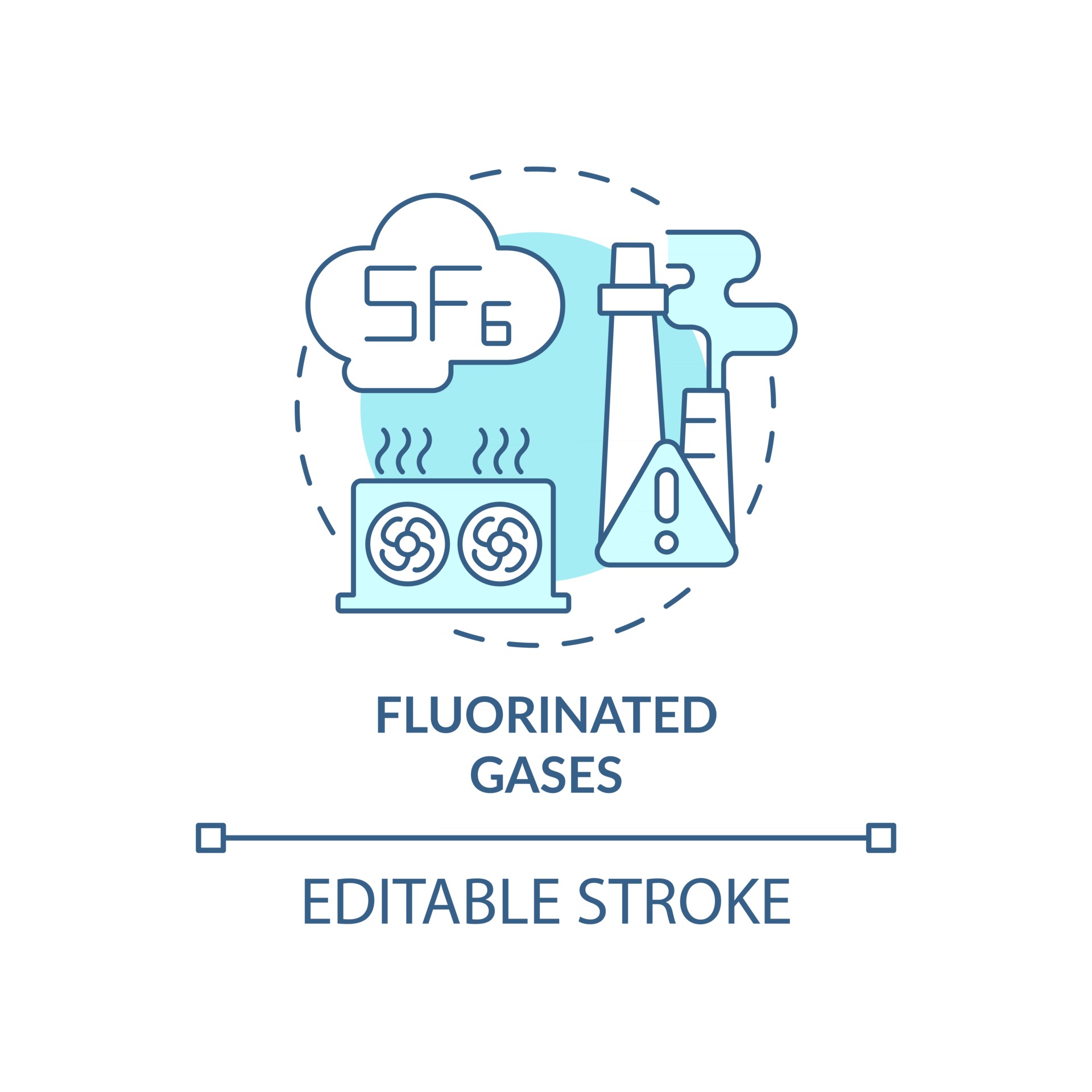This is a detailed diagram depicting the flow of fluorinated gases. At the bottom, bold text reads "EDITABLE STROKE," colored in dark teal. Above this text, a horizontal line stretches across, flanked by two squares on either end. Moving upwards, another bold label says "FLUORINATED GASES."

The central part of the diagram features a navy-blue dashed circle, containing a detailed illustration. Inside this circle, there's a factory with chimneys emitting gas, alongside a large home air conditioning unit, marked with "SF6" in a cloud-shaped figure. Nearby, there are beaker-like structures with light blue lines suggesting emitted air. An additional element within this circle is a triangular warning symbol with an exclamation mark, possibly indicating caution or importance.

The dashed line within the circle follows a clockwise path, connecting these various elements and returning to the SF6 cloud, creating a continuous loop that visually represents the cycle of fluorinated gases.